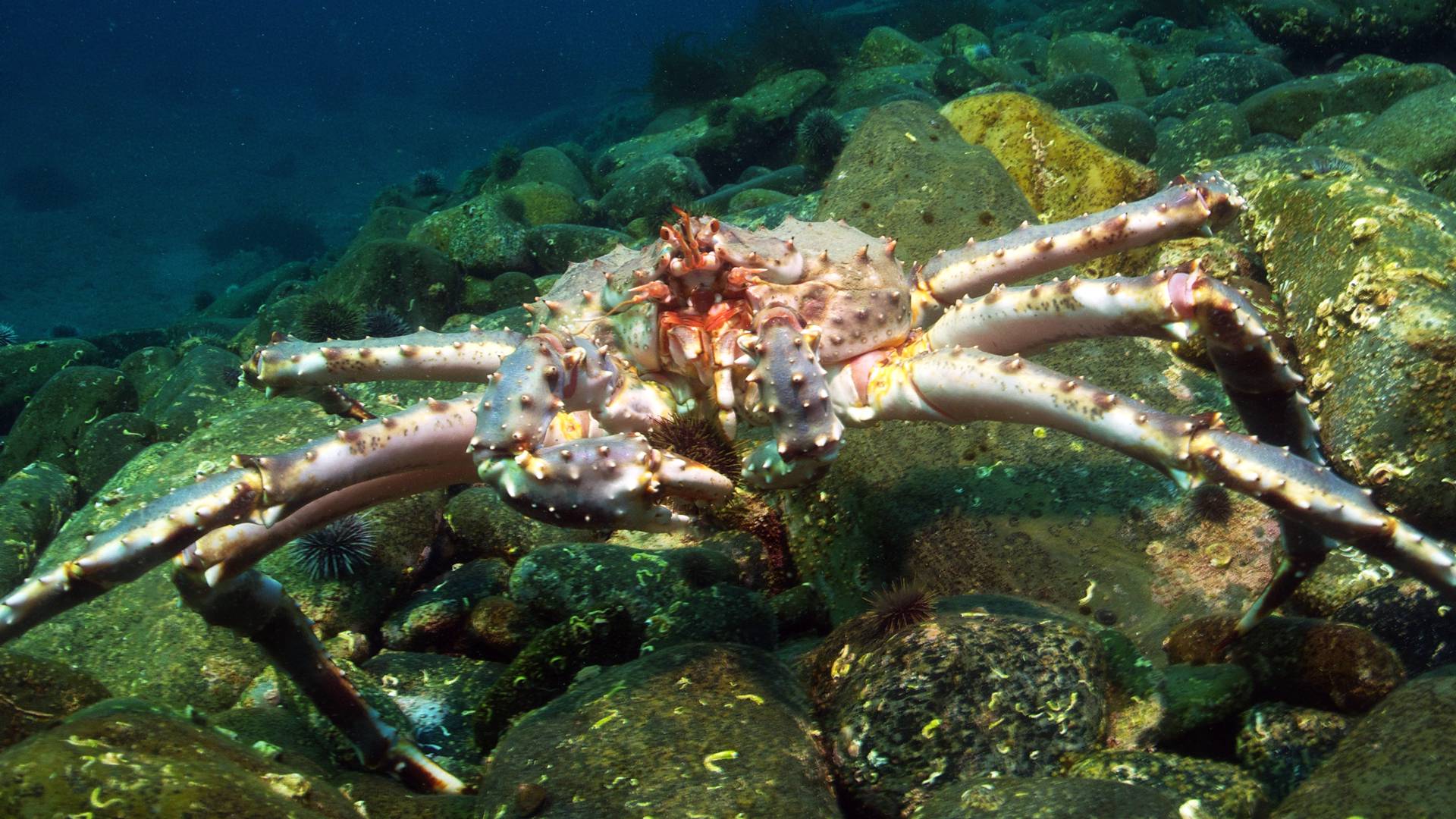This detailed underwater photograph captures a striking close-up of a large king crab standing on a bed of rocky terrain. The crab's silvery white and blue-tinted legs, adorned with small spikes, are prominently displayed, bent at their joints and extending outwards, with some resting on the moss-covered, greenish rocks below. The crab's body displays a mix of blue, white, and golden hues, with a notable red spot at its center and orange tentacle-like projections near its mouth and eyes. The creature appears to be consuming an anemone, which it holds in its front claw. The surrounding underwater environment features a mixture of green-tinted rocks, possible fungal growths, and darker blue water in the background, adding depth and contrast to the image. This captivating photograph showcases the intricate details and vivid colors of the crab and its aquatic habitat.